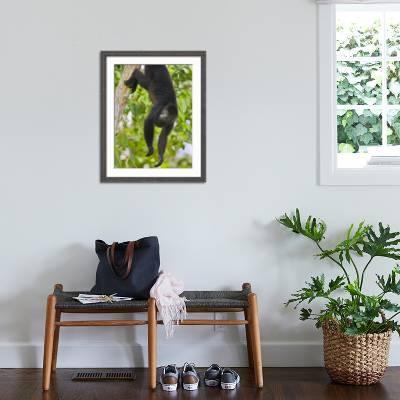The image depicts a room with light gray walls and a simple, yet organized setup. Dominating the lower central part of the image is a wooden bench with a gray cushioned seat, visible through its three sturdy legs. The bench serves multifunctional purposes; underneath, it holds two pairs of shoes—one brown and one grayish-green. On top of the bench, a dark blue tote bag rests beside a white shawl, while a paper is also visibly placed there. To the right of the bench stands a potted houseplant in a wicker basket, its green leaves reaching toward a window partially visible in the upper right corner, showing some greenery outside. Above the bench, a framed photograph captures attention with its thick white border and a thinner black frame around what appears to be an image of a dark-colored monkey, with surrounding greenery. The room’s floor is dark wood, and an air vent for an AC and heating unit is partially visible under the bench, in addition to the shoes. The composition of the image creates a cozy and functional entryway or small sitting area within the room.